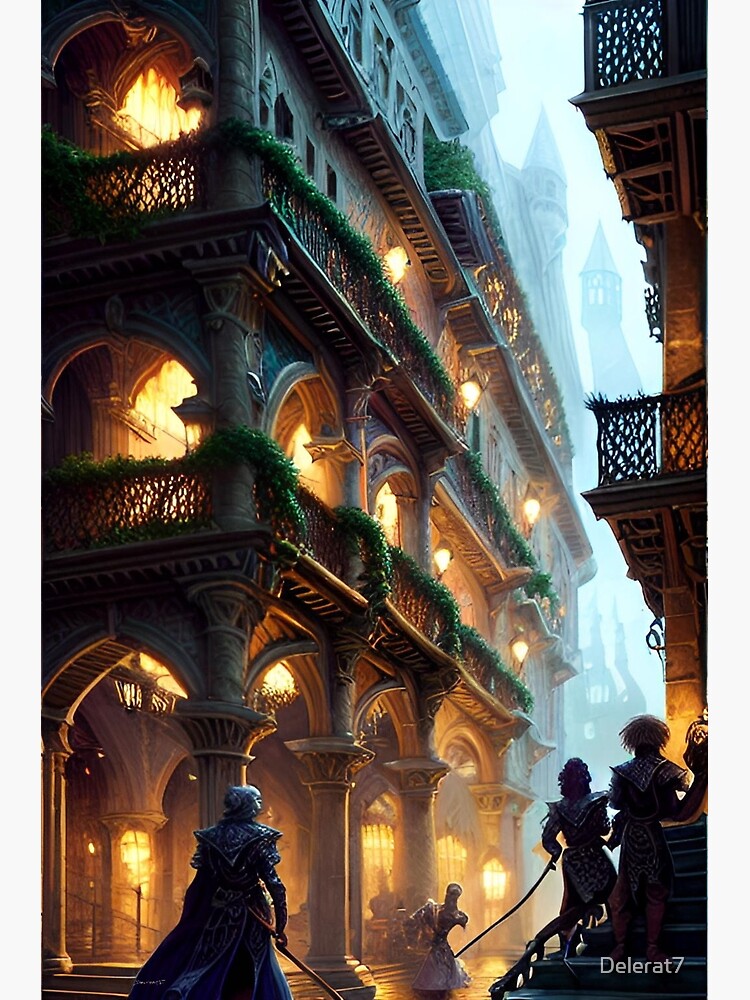In this vivid screenshot from a fantasy video game, we are drawn into the medieval ambiance of an elven cityscape. The scene is set in a narrow alley flanked by two impressive three-story buildings adorned with balconies draped in lush green ivy and illuminated by ancient gas lamps. The building on the left, dominating much of the frame, features large white marble columns and multiple stories that lead up to intricately crafted steeples with sharply pointed, dart-like roofs. 

Amidst this backdrop, a dramatic confrontation unfolds. On one side, three armored men, brandishing swords and sticks, stand alert, prepared for battle. Their stance and demeanor convey readiness and vigilance. Opposite them, a woman in a flowing white dress appears startled and uncertain. Beside her, a younger lady clad in pink ascends the steps of the adjacent building, her face obscured.

The scene is further enriched by details hinting at an impending conflict. A skeletal figure is splayed in the middle of the street, seemingly the focus of the men's attention. The intricate environment and atmosphere are capped off with a signature in the bottom right corner, reading "DELERAT 7" in white text, marking the artwork with a personal stamp.